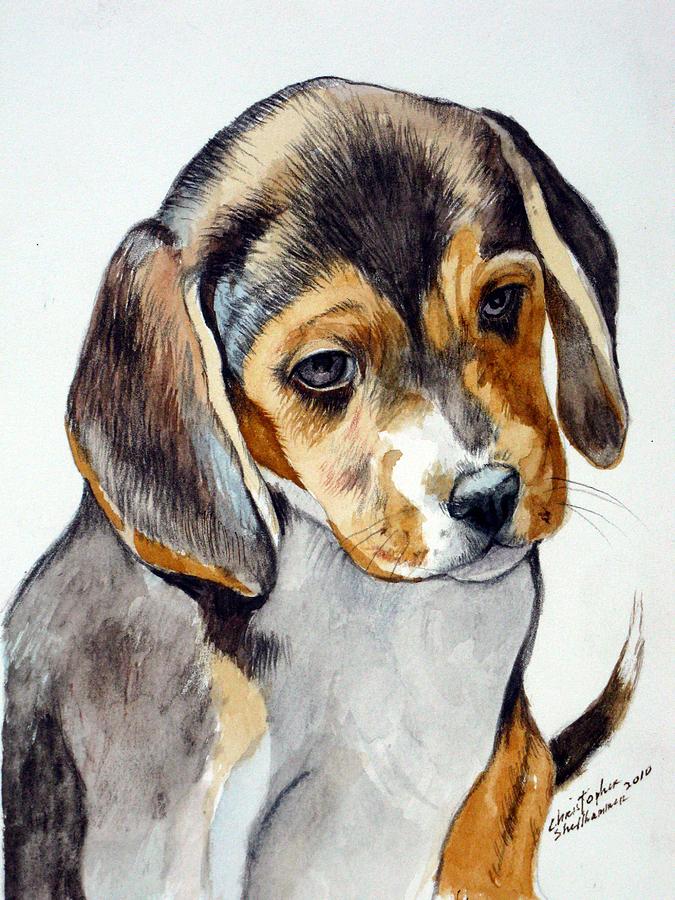This is a detailed and colorful illustration of a young beagle puppy. The background is predominantly light grey, providing a subdued contrast to the puppy's vibrant coat. The puppy's head is crowned with dark fur, transitioning into a lighter golden brown around its eyes and cheeks, punctuated by a white muzzle and snout near its black nose. Its expressive brown eyes and downward gaze impart a sad expression as it looks downward to the right. The floppy ears, a blend of black and muted golden tones, hang endearingly by its head. The pup's body features a mix of black and grey, with a golden tinge visible on parts of its back, and a white chest that stands out against the darker hues. Only a portion of its black tail, tipped with greyish white, is visible, poking from the bottom right corner of the image. The detailed artwork is signed by the artist in the bottom right corner with "Christopher Shellhammer, 2010" inscribed, though part of the signature is slightly illegible.